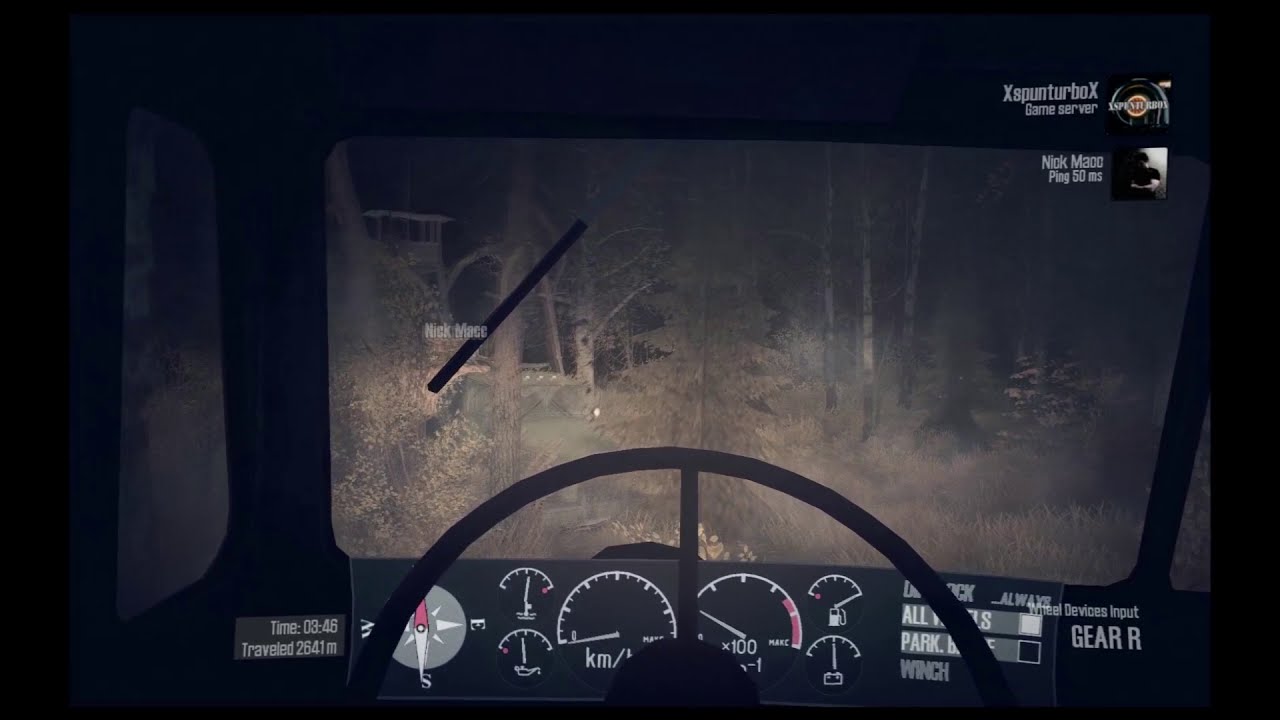A high-resolution screenshot of a video game showcasing a gritty, textured 3D environment. At the forefront, there is a black smart steering wheel adorned with multiple gauges including a compass, gas, battery, fuel, and speed indicators. The perspective immerses the viewer into a first-person view from inside a boxy vehicle, driving through a dense, dark forest with tall, mixed evergreen and deciduous trees visible through the windshield. In the upper part of the image, the game server information is displayed, showing "X-Spun Turbo X game server" and the player "Nick Mao" with a ping of 50MS, represented by a profile picture of a person with crossed arms wearing a black short-sleeve shirt. The user interface features additional text, notably "Unreal devices input gear R" at the bottom right and "time 0446, travel 2641M" at the bottom left, emphasizing the in-game time and traveled distance. The left-hand side of the dashboard shows other controls and information like "all" and "park" with possible winch functions, enhancing the sense of an interactive and detailed gaming experience.